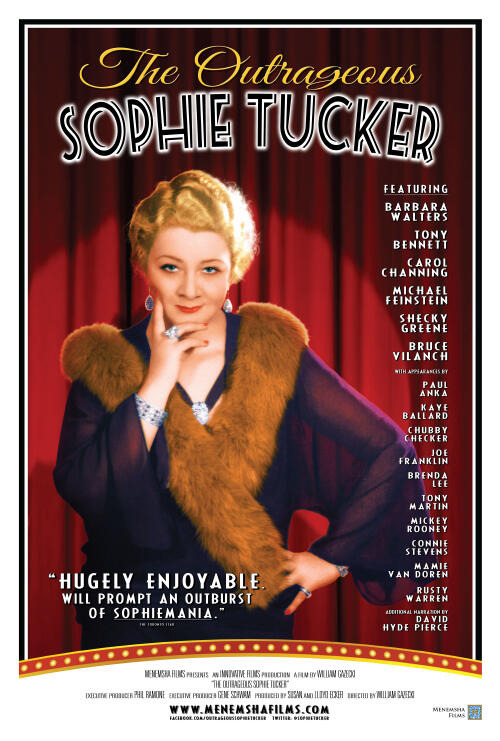The poster depicts a movie titled "The Outrageous Sophie Tucker." At the top, in yellow italic writing, it says "The Outrageous," followed by "Sophie Tucker" in bold black and white text that appears illuminated in 3D. Dominating the left side of the poster is an image of Sophie Tucker, a rich-looking woman with short, blonde, wavy hair styled in an old Hollywood fashion. She stares directly at the viewer with blue eyes, red lips, and red-painted nails. Sophie wears a luxurious dark blue or purplish dress or jacket lined with thick brown fur, which drapes from her left shoulder to her right. Her right hand touches her face, with two fingers on her cheek and the rest under her chin, showcasing her elaborate silver jewelry, including a large ring, a bracelet, and teardrop earrings. Behind her hangs a traditional red theatre curtain, draped and spotlit.

Running down the right side of the poster are names of featured personalities: Barbara Walters, Tony Bennett, Carol Channing, Michael Feinstein, Shecky Greene, Bruce Villance, with additional appearances by Paul Anka, Kay Ballard, Chubby Checker, Joe Franklin, Brenda Lee, Tony Martin, Mickey Rooney, Connie Stevens, Mamie Van Doren, and Rusty Warren, along with an additional narration by David Hyde Pierce. At the bottom left, a testimonial reads, "Hugely enjoyable, will prompt an outburst of Sophie-mania." The poster is bordered by a white and black frame, with a URL at the very bottom indicating "www.menemshafilms.com."